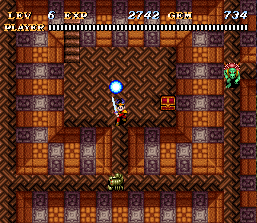In this intricate scene from a computer game, the central character is depicted wielding a majestic sword, poised beside a luminescent globe of white and blue hues. Nearby, a tantalizing treasure chest awaits discovery, nestled within the heart of this chamber. The chamber itself features multiple winding paths that twist and turn, forming a labyrinth of danger and opportunity. Various menacing creatures patrol these paths, guarding the treasure jealously. Among them is a creature resembling a scorpion, menacingly positioned close to the entrance. Another formidable opponent, with a massive green head and equally enormous arms, prowls nearby. Both creatures add a layer of peril for the player, who must navigate these dangerous routes. Along the top of the game screen, several indicators provide vital information, including the current game level, helping the player strategize and progress through this captivating quest to seize the treasure and escape unscathed.